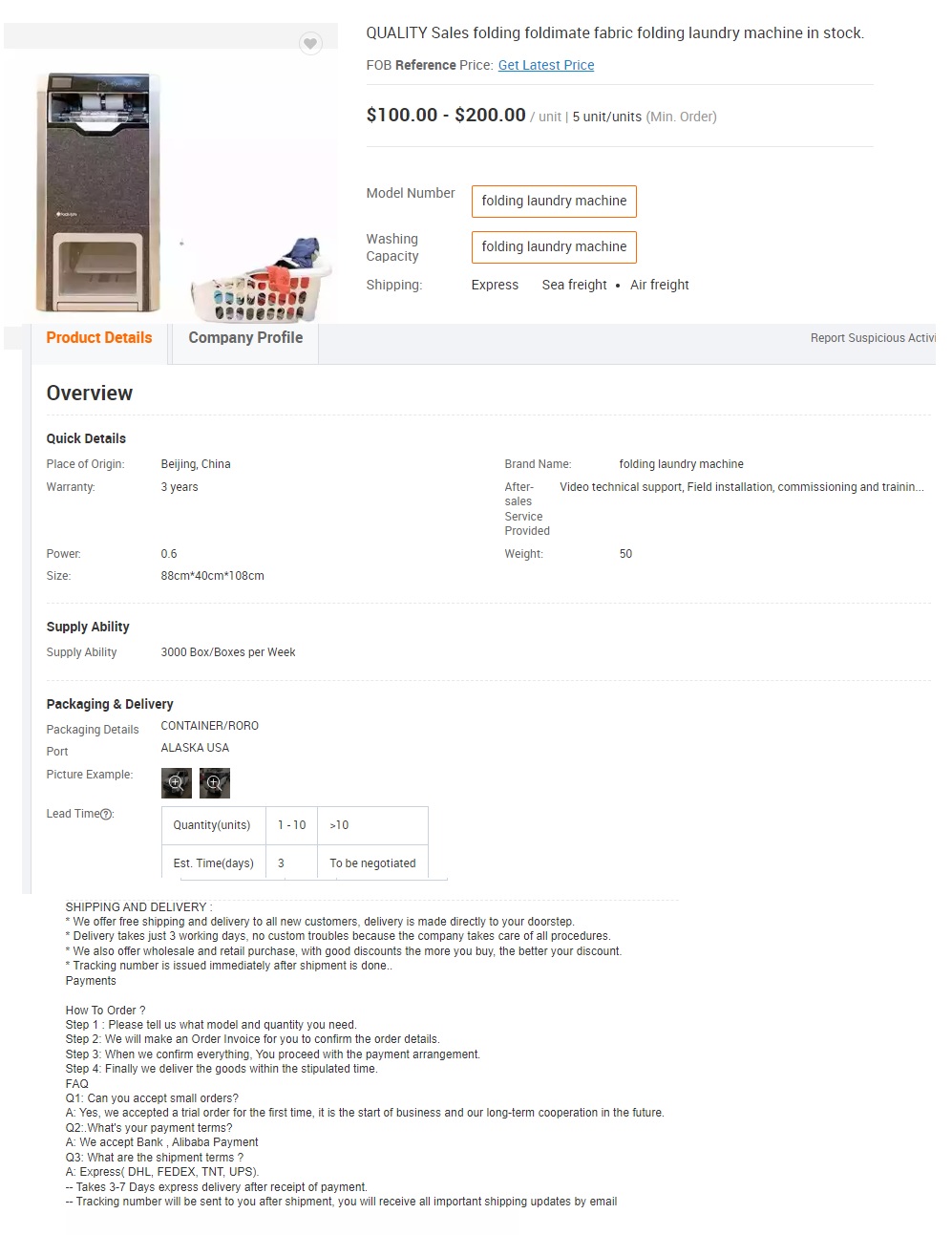Screenshot of a website displaying a product available for purchase: a "Quality Sales Folding Foldamate Fabric Folding Laundry Machine," currently in stock. The price ranges from $100 to $200 per unit. On the left side of the screenshot, there is an image of the machine, which resembles a washing machine, accompanied by a laundry basket. Although the specific functions of the machine are not immediately clear, it is implied to fold laundry. The product is manufactured in Beijing, China, and comes with a three-year warranty. Below the main description, there is a list of detailed product specifications in black text, which includes information on shipping and delivery directly to your doorstep, although much of this text is difficult to read due to its small size.